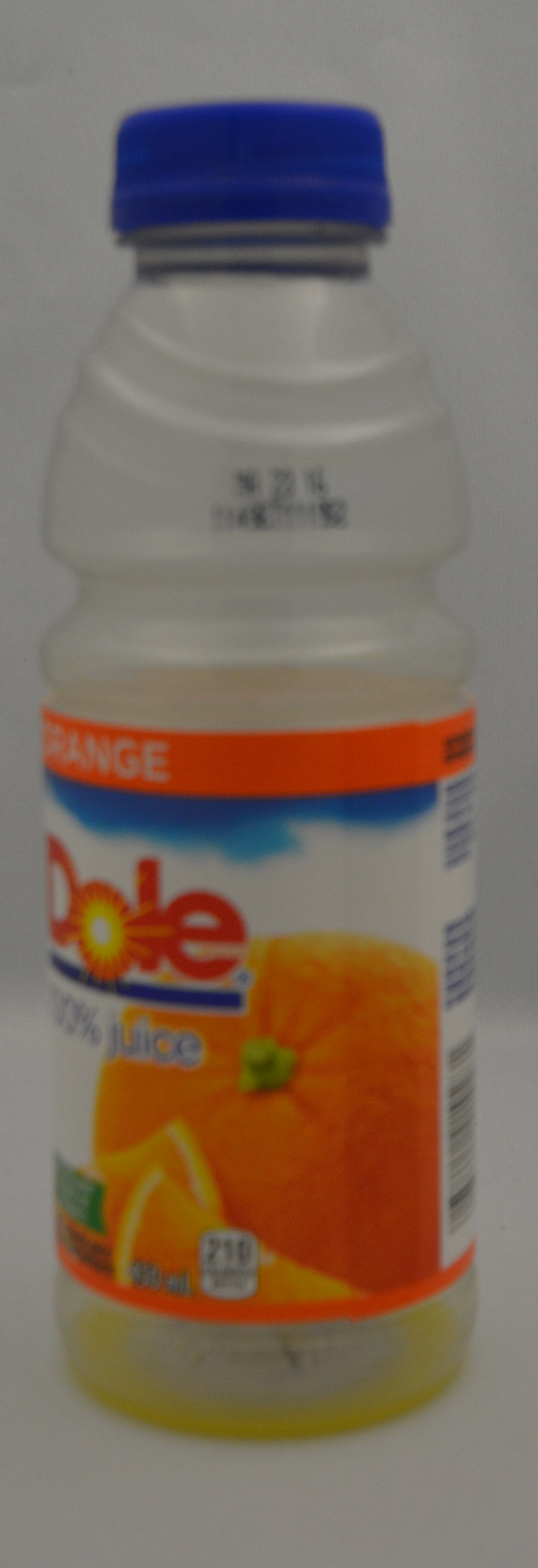The image shows a slightly blurred plastic bottle with a twist-off blue cap. A small amount of orange-colored liquid remains at the bottom of the bottle, suggesting it originally contained more of this fluid. The bottle is positioned so that its expiration date, printed on the label, faces directly towards the camera. The front of the bottle label is partially visible to the left side of the image. The label appears to be from the brand "DOLE," and features an illustration of a whole orange with its stem, accompanied by a few orange slices.